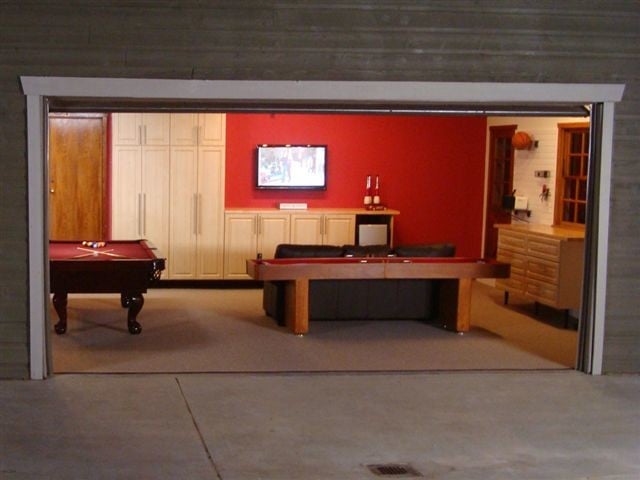This image depicts a transformed garage, now serving as a well-appointed man cave. The garage door is open, framed by a thin white border and flanked by gray siding. Outside, there is a gray concrete driveway, leading into a carpeted interior with a light gray carpet. Inside, the left side features a dark wooden pool table with a vibrant red felt top, set against a painted red wall. A flat-screen television is mounted on this wall, above a series of short, cream-colored cabinets, with taller cabinets located to the television's left. There are also wine bottles on one of the counters, hinting at a bar setup.

Across from the television, there's a comfortable brown sofa, with a wooden table stand positioned behind it. Additional details include another pool table with a black felt top located behind the sofa, and a possible foosball or air hockey table. The garage also contains a brown door to the left and another door to the right, where a basketball is visible hanging on the wall. A brown drawer is situated on the right side, next to the right door. The converted space has elements of leisure and entertainment, clearly designed as a man cave.